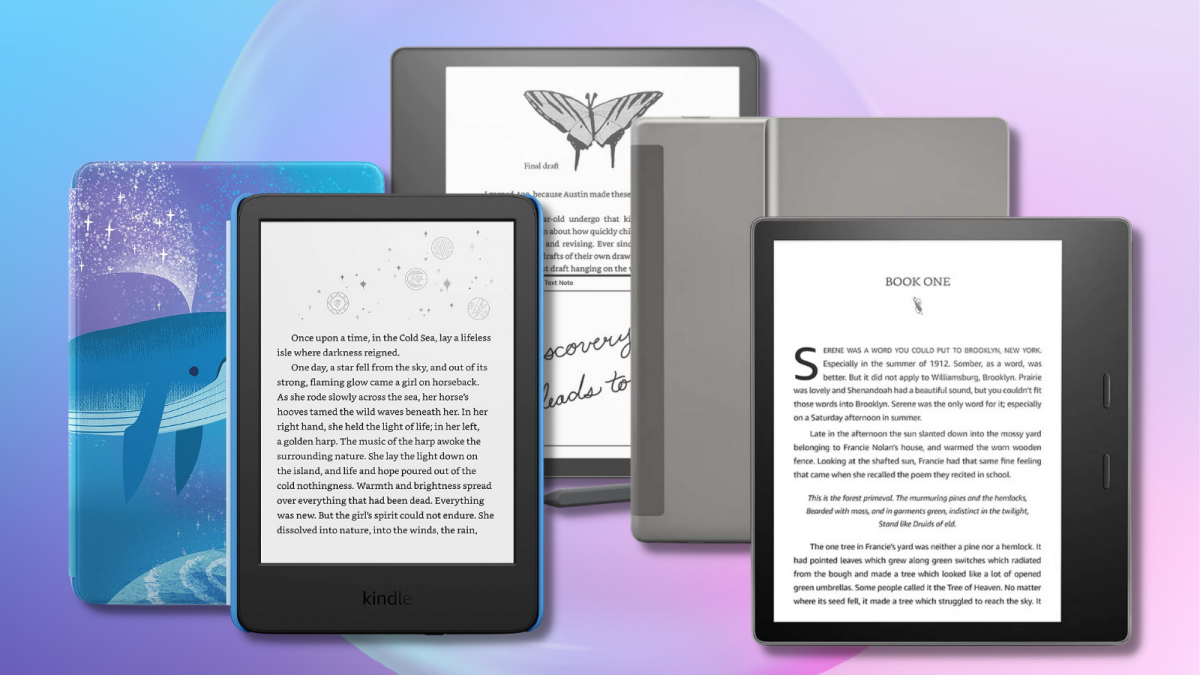The image features a collection of five different e-readers and their cases against a vibrant, computer-generated background blending shades of blue, purple, and pink with a bubbly design. On the far left, an e-reader encased in a cover displays an artistic image of a cartoon whale expelling sparkles, set against a matching gradient background. Directly to its right, another e-reader with its cover folded back reveals the device partially overlaying the whale design. In the middle, an e-reader displays text and a butterfly design, standing slightly recessed behind the others. To the right of this is a larger tablet with a prominent gray cover, obscuring part of the butterfly e-reader. The final device, in the foreground on the right, is another large e-reader, characterized by a dominant black right column and a visible book text. All e-readers are black or gray, contrasting sharply with the colorful, dynamic background.